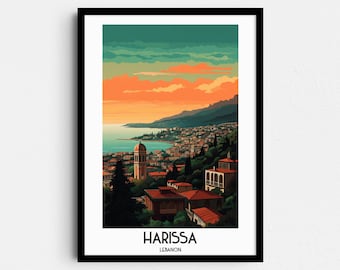This photograph captures a framed print of moderate resolution, possibly taken with a low-resolution camera, which impairs some finer details. The frame is black, possibly lacquered, and contains a white border within it. The wall it hangs on is a light, slightly off-white or gray color. The print depicts a picturesque coastal city, identified by the text "Harissa, Lebanon" at the bottom in black font, though a smaller, illegible word also appears.

The imagery within the print showcases a vibrant coastal city characterized by numerous red-roofed and white buildings. A prominent tall building stands out among the structures. The cityscape extends to the water's edge, with either a large lake or the ocean visible on the left side. To the right, mountains rise up from the water's edge. The sky above transitions from warm oranges and yellows at the horizon, blending into darker shades of blue higher up, interspersed with clouds. The entire scene is bathed in the hues of a setting sun, casting a serene light over the landscape.